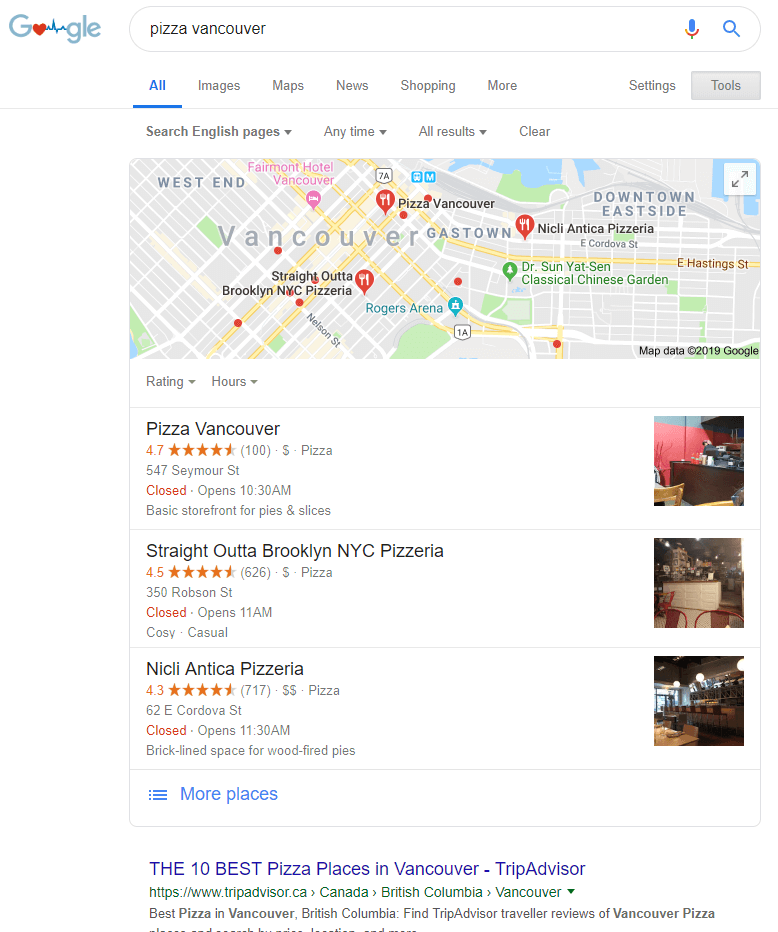A Google Maps search for "pizza in Vancouver" displays various results, including images, maps, news, and shopping options. The search prominently features a map highlighting different pizza establishments across Vancouver. 

The first result is "Pizza Vancouver," rated 4.7 stars. The establishment, which opens at 10:30 a.m., has a basic storefront offering pies and slices but is currently closed.

The second result is "Straight Outta Brooklyn NYC Pizzeria," boasting a 4.5-star rating. This cozy and casual venue opens at 11:00 a.m. but is also currently closed.

The final highlighted pizzeria is "Nicli Antica Pizzeria," with a 4.3-star rating. Known for its brick-lined space and wood-fired pies, it opens at 11:30 a.m. and is presently closed as well.

Beneath these results, there is a section listing the "10 Best Pizza Places in Vancouver," sourced from TripAdvisor.